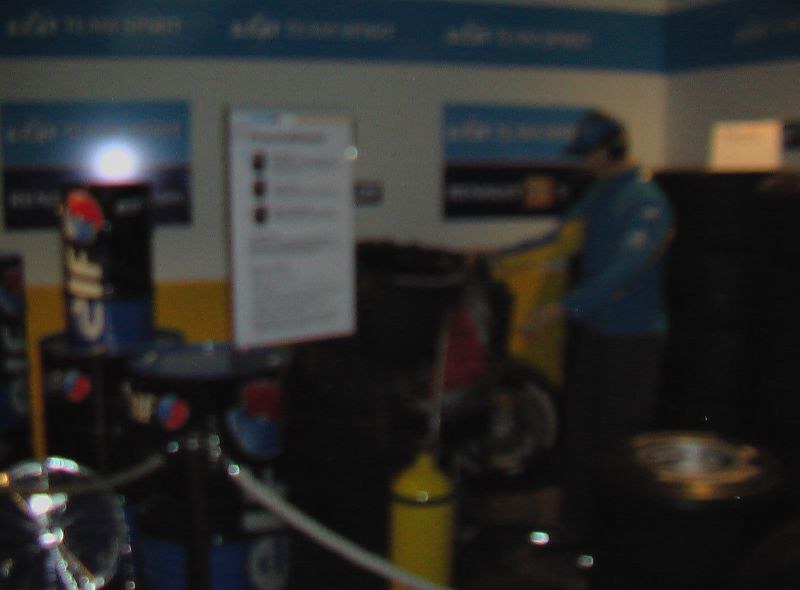This color photograph, although dimly lit, blurry, and out of focus, depicts an indoor scene that appears to be inside a garage. The grey wall in the background features a blue stripe along the top with some unreadable white writing on it. Central to the image is a large rectangular sign displaying black writing and bullet points arranged down the middle, with additional text to the left and below the bullets. 

Surrounding this main sign, there are two smaller signs with blue tops and black bottoms, both inscribed with white text. To the right, a person is visible, identifiable by their hat, and clothing including a blue top and dark trousers. They are positioned in front of a yellow object. 

In the foreground of the image is a yellow canister located centrally, with a black object adjacent to the main sign. The bottom left corner of the image includes some metallic items resembling cans, jars, or potentially motor-related objects. 

The scene is further illuminated by varying light sources: a yellow light and a white light directed at a blue sign on the left-hand side, and a small illuminated rectangle emitting a softer yellow light in the upper left corner. Otherwise, the overall image remains quite dark.